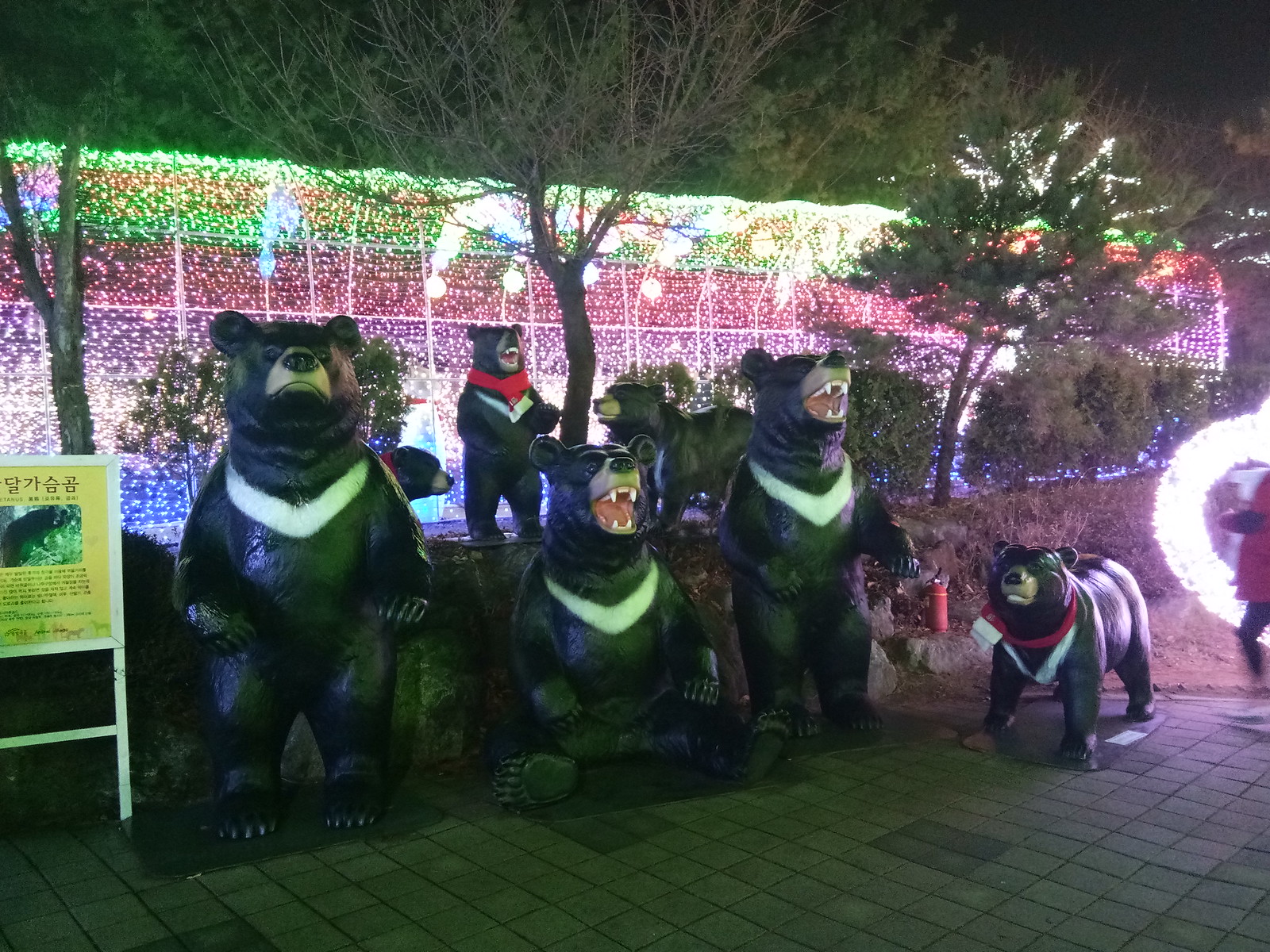This detailed night-time photograph captures a whimsical display of bear statues, likely made of plastic or cement, amid a festive setting. The scene features six bears, each with a distinctive white v-shaped stripe across their otherwise dark brown, almost black fur. Three of the bears stand upright on their hind legs with their mouths agape in a menacing expression, while one is seated in a human-like pose, and two, including a smaller one, are positioned on all fours. The bears are arranged on elevated rectangular bases placed on a surface mimicking granite or brick paving. The background showcases a vibrant array of Christmas-like fairy lights in hues of green, red, blue, purple, white, and orange, casting a colorful glow over the setting. Silhouettes of trees stand against the backdrop of lights enhancing the festive atmosphere. To the left of the bear statues, a white-framed sign displays an image of the bears with text and a header in what appears to be Japanese or Chinese.